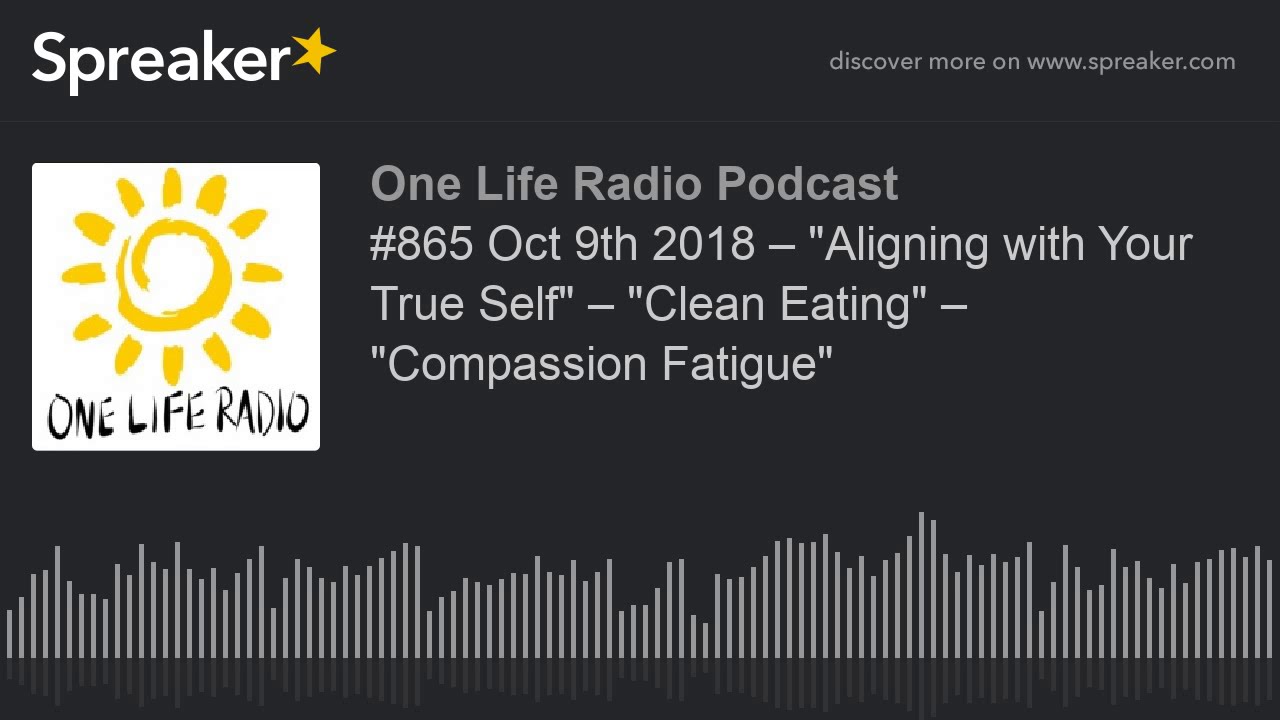This image provides intricate details about a podcast against a black background. Positioned at the top left is the text "Spreaker" followed by a yellow star, serving as a logo. At the top right, the text reads "Discover more on www.Spreaker.com." Beneath this, on the left side, there is a white square featuring an outline of a yellow sun with the text "One Life Radio" beneath it. Central to the image are the words "One Life Radio Podcast #65, October 9th, 2018 – Aligning with Your True Self, Clean Eating, Compassion Fatigue." At the bottom, a series of vertical white lines of varying heights resemble sound waves.